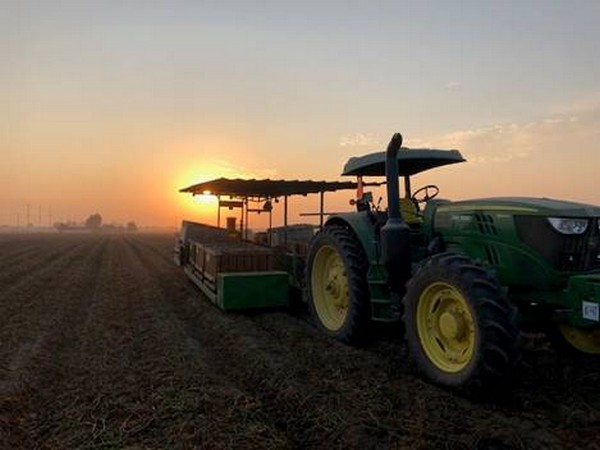In this atmospheric photograph taken during either sunrise or sunset, a giant John Deere tractor, characterized by its iconic green paint and yellow wheels, stands prominently in a vast, freshly tilled field. The tractor is facing us and turning slightly to the left, pulling a trailer or some sort of agricultural machinery that appears to be responsible for the neat, endless rows of soil stretching as far as the eye can see. The low sun casts a dim, pinkish-red and blue hue across the hazy sky, with the horizon glowing softly. In the far distance to the left, the faint outlines of a barn or silo and some telephone poles are just visible, adding to the tranquil, rural scenery. The terrain and machinery are subtly cloaked in a light fog or smoke, giving the image a surreal and ethereal quality. The tractor, though detailed with features such as a yellow seat, black roof, and steam pipe, appears unmanned and stands alone in the vastness of the farmland.